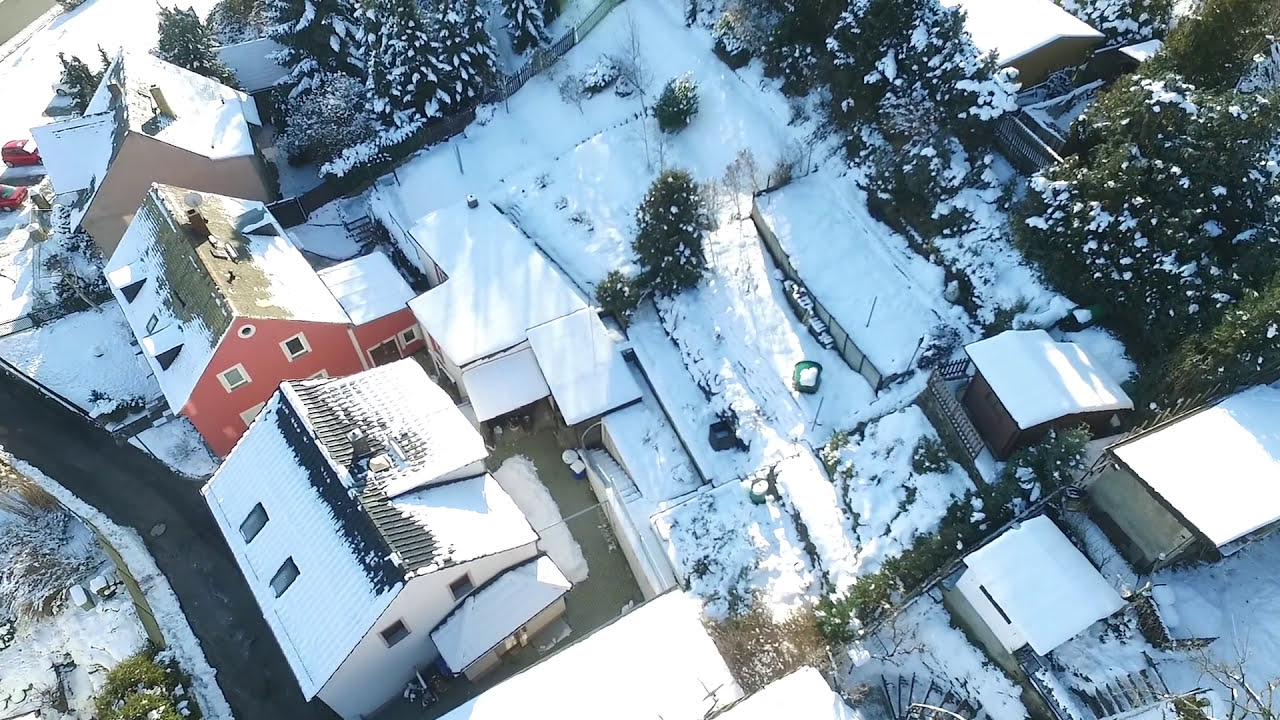This high-altitude aerial photograph, likely captured from an aircraft or drone at approximately 200 feet, depicts a snowy daytime scene of a neighborhood. The clear blue sky suggests it was taken in the later part of the day, with bright light illuminating the landscape below. 

In the image, a patchwork of snow-covered rooftops and backyards dominates the scene, with the snow varying in depth but presenting a fairly consistent blanket across trees, roofs, and ground. The left side of the photo features a relatively clear road, running beside three distinctive houses arranged in a line: a beige house near the top, a red house in the middle, and a white house at the bottom.

To the right, multiple smaller structures, including sheds and potentially a barn, are scattered amidst the snowy landscape, their roofs burdened with snow. Pine trees and other foliage are visible both to the right and across the top of the image, snow clinging to their branches. The image captures the encompassing quiet and stillness of the snowfall, with features like a shoveled driveway standing out amidst the otherwise undisturbed snow cover. This detailed view provides a comprehensive look at the serene yet dynamic arrangement of this wintry neighborhood.